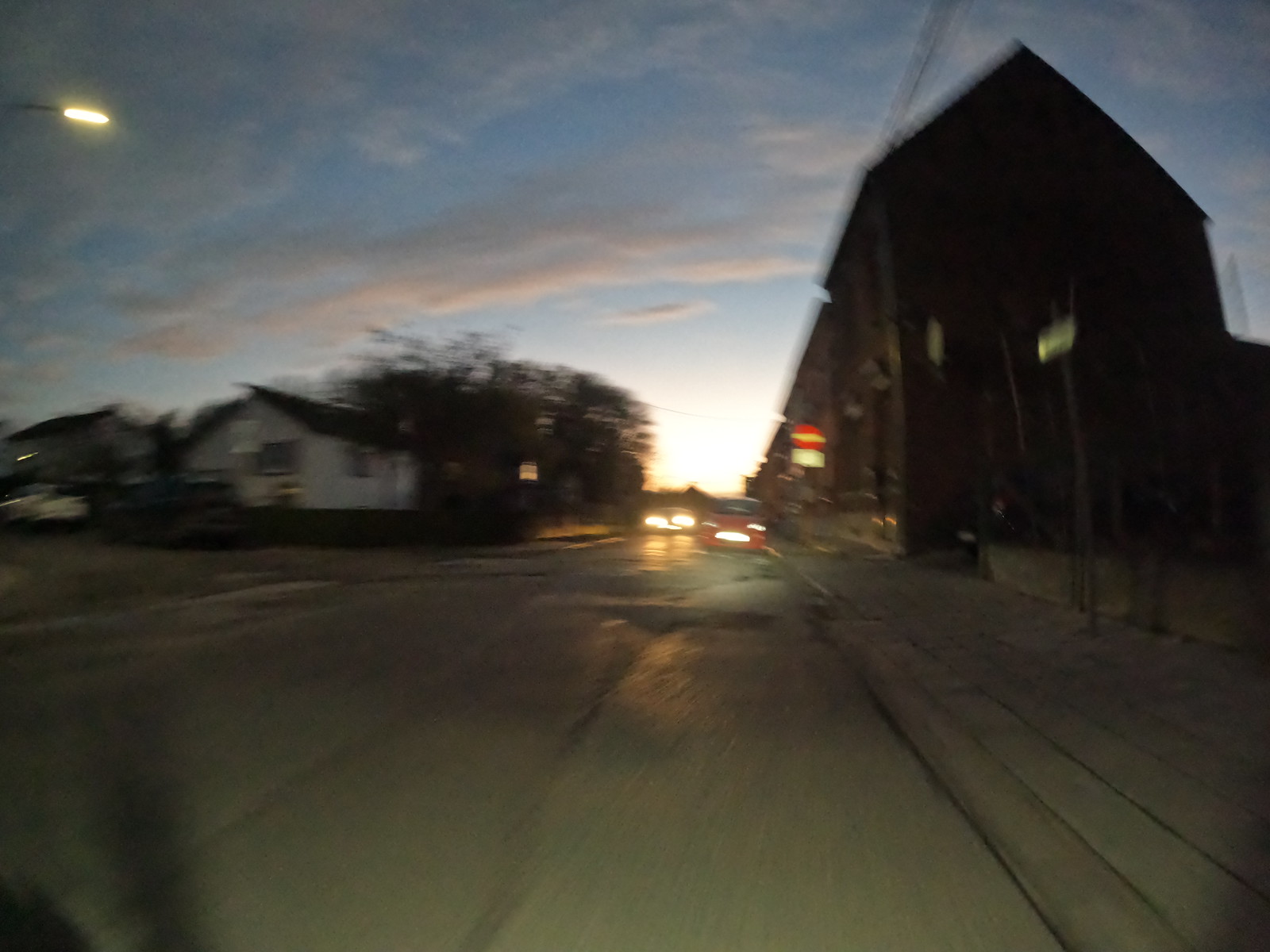The photograph captures a blurry street scene taken around sunset or dusk from the perspective of someone driving in a car. The sky transitions from a mellow blue to a bright orange at the center, amidst wispy clouds. The street, primarily occupying the foreground, features a red car parked on the right side, next to a building with a lit sign, and another car driving towards the viewer with its headlights on. To the left of these cars, a bunch of trees can be seen. Residential houses line both sides of the street, with a row of buildings on the right. A streetlamp, with its light on, peeks from the top left of the image. The sidewalks, one on each side of the street, are distinctly visible, with the right one featuring bricks laid in it. Furthermore, a stop sign is noticeable on the street, reinforcing the small-town ambiance suggested in the image.